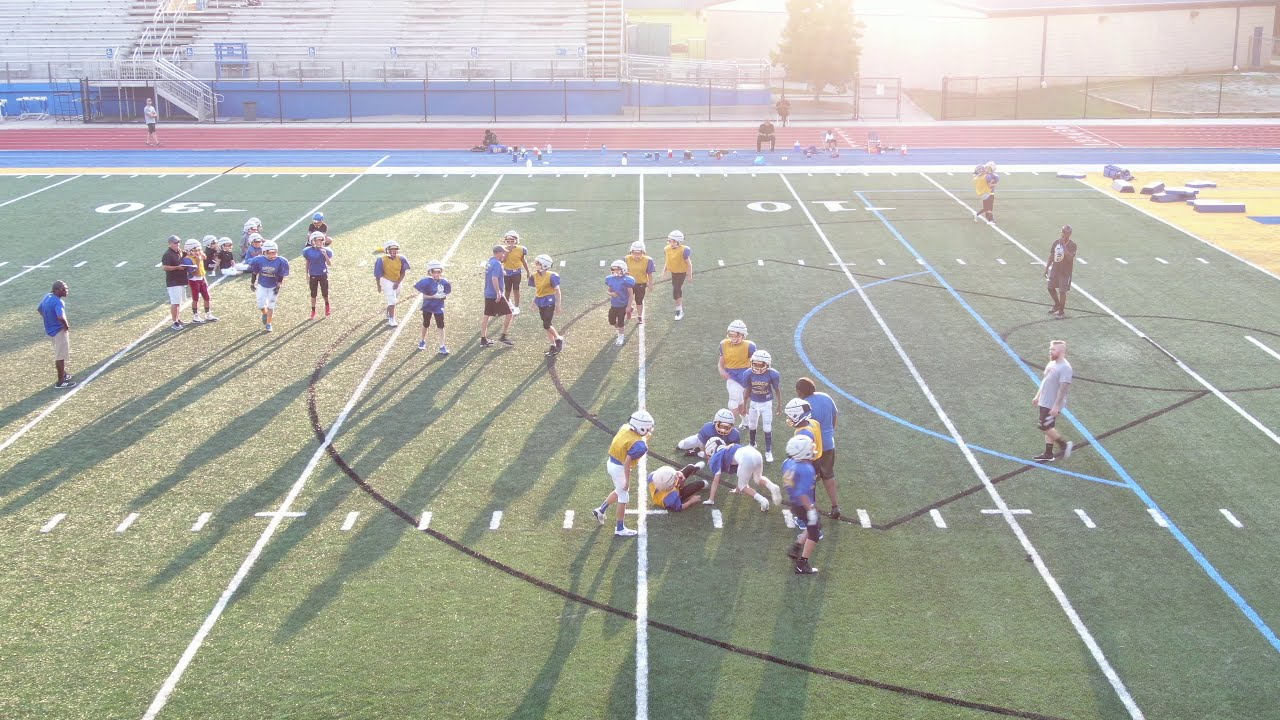This image captures a youth football practice session on a well-marked football field. Most of the field, stretching from the 30-yard line to the goal line, is visible, with key yard markers like the 30, 20, and 10-yard lines clearly identifiable. The young players, likely aged 12 to 14, are distinguishable by their smaller stature and are equipped with blue shirts and white helmets. Some players wear additional yellow pullovers over their blue shirts, indicating a scrimmage practice. Adults in shorts and t-shirts, presumably coaches, are interspersed among the players, overseeing the practice. The coaches are identifiable by their attire: one in a gray t-shirt and black shorts, another in a black shirt, and a third in a blue shirt and tan shorts. In the background, a red running track encircles the football field, leading up to steel gray bleachers supported by a blue wall. Spectators can be seen behind the fence that borders the track, adding a sense of community involvement. The early morning or late afternoon sun casts long shadows of the players across the green field, emphasizing the time of day during this vibrant youth practice session.